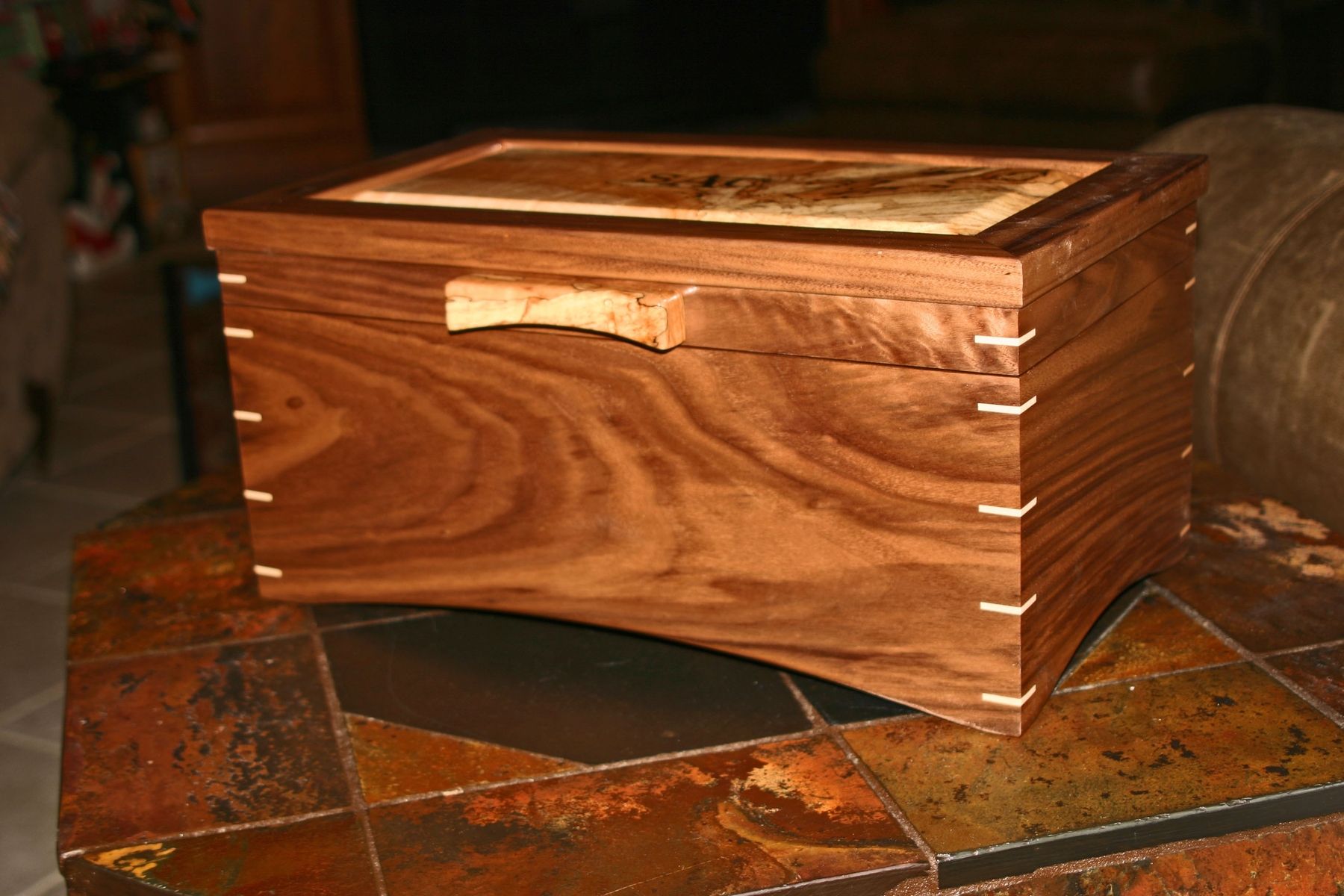The image displays a wooden trunk crafted from dark brown wood with a pronounced wood grain marbling. The trunk features a lighter-colored handle on its lid, suggesting it's a functional storage item. Notably, the trunk is adorned with five light-colored reinforcement strips—possibly made of a lighter wood or ivory—on each corner, running the length of the trunk from the lid to the base. These reinforce and accentuate the corners, adding both strength and decorative contrast. The chest is situated on a tiled floor, which appears to consist of multicolored tiles in shades of dark red, yellow, and orange. The detailed craftsmanship and practical design suggest that this trunk could serve as an ideal container for storing jewelry, keys, sunglasses, or other small items.